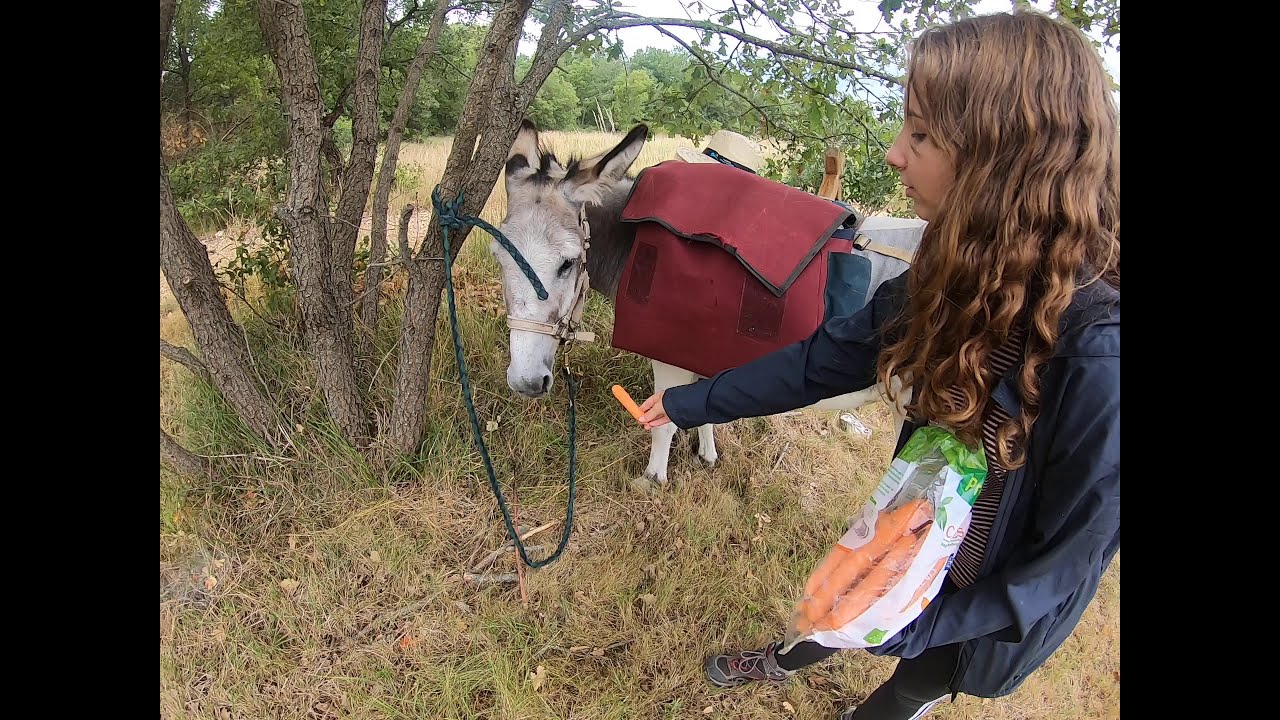In the center of the image, a beautiful white burro with black and brown accents on its ears and forehead lock stands tied to a scrubby oak tree with a green rope. The burro is carrying a large burgundy backpack with a blue pocket on one side. Adjacent to the burro, a young teenage girl with beautiful skin and long, wavy brown hair is feeding it a carrot from a large bag she holds in her left hand, while offering a carrot with her right hand. The girl is wearing a dark blue jacket over a blue and white striped shirt, paired with pants and tennis shoes. The setting appears to be at the edge of a field in late summer, as indicated by the tan, dry grass with sparse patches of pale green. In the background, a tree line suggests a nearby forest. Additionally, there is a hat visible on the opposite side of the burro, which might be attached to or resting on it. Framing the image are black rectangles on the left and right sides.